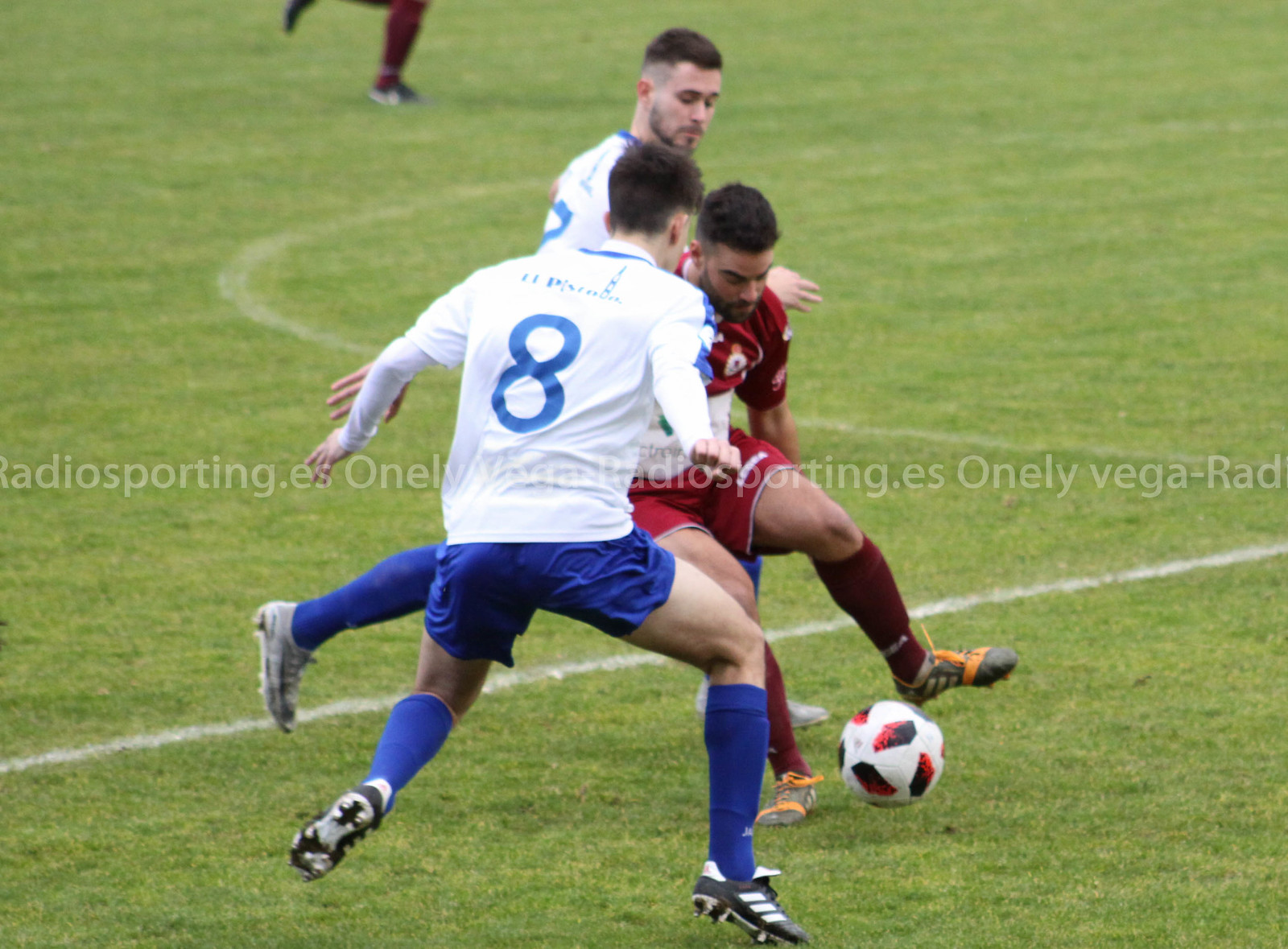The full-color photograph captures an outdoor daytime soccer match on a green football pitch. It prominently features three male players and part of a fourth player's legs. The players are engaged near the midfield with visible white chalk lines on the grass. One player, identifiable by his number eight jersey, has his back to the camera. He has short brown hair and wears a white shirt with blue shorts and blue socks, paired with black and white cleats. In front of him, a player in a red kit, including red socks and black and orange boots, is in possession of a slightly unusual white soccer ball adorned with black and red markings. Another player in the same white and blue kit is positioned nearby. In the background, only the shins and feet of another player in a red kit are visible, indicating their approach towards the play. A watermark reading "radiosporting.es" is faintly visible across the image.